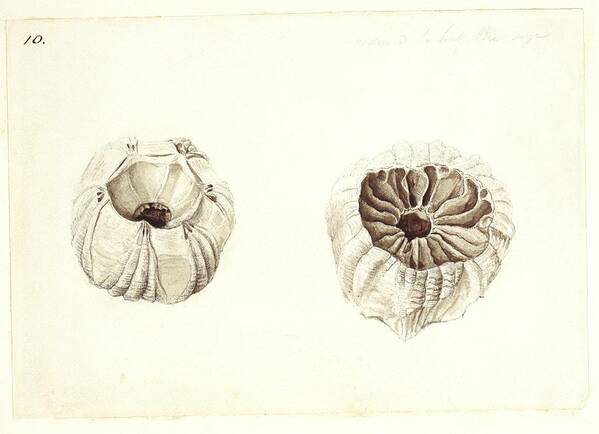This detailed caption summarizes the descriptions cohesively:

The image depicts a detailed black and white sketch on off-white, parchment-like paper, resembling an old illustration from a nature book or museum catalog. In the top left corner, the number "10." is inscribed, with faded, unreadable handwriting in the upper right. The artwork consists of two versions of a similar, unidentified object, perhaps a crustacean or a peculiar shell-like organism.

On the left, the object appears circular with a crater-like opening at the top, leading into a smaller hole, reminiscent of a closed pouch or an unaged, intact specimen. Its surface is a muted beige and off-white, with no vibrant colors. To the right, the object is depicted as if it's been cut open or aged, revealing complex, web-like structures or fleshy, compartmentalized pockets, similar to an opened duffel bag or a dried-out, sliced fruit. This side seems like the interior view, showcasing detailed textures and internal organization. The overall impression is of an ancient or alien-looking find, rendered with pencil-like precision, and possibly part of a nature study or fossil illustration.